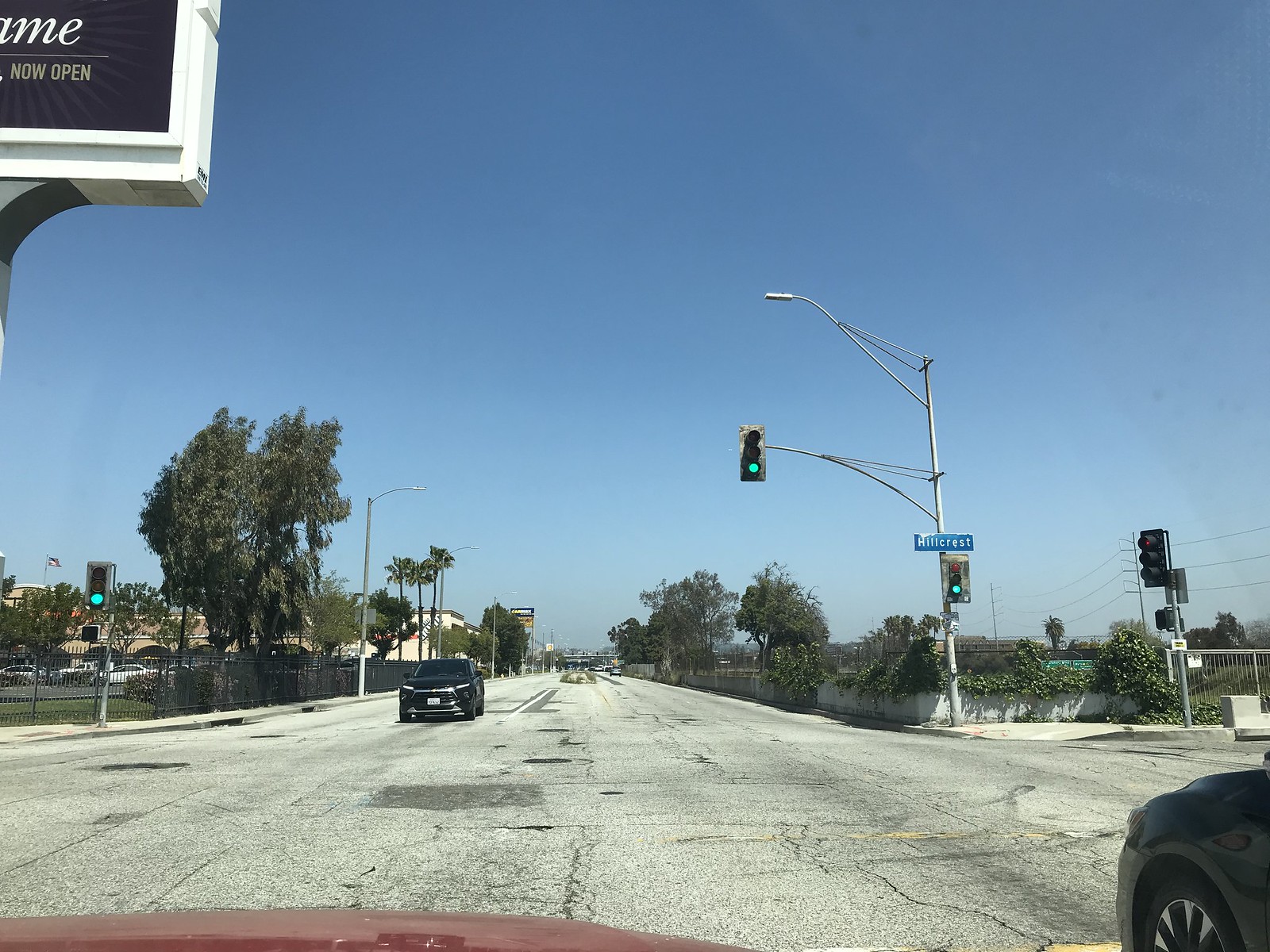This photograph, seemingly taken from inside a vehicle, captures a vibrant street scene at a four-way intersection. The lower right corner of the image reveals a portion of the photographer's red car, while next to it, a dark-colored station wagon—possibly dark gray or dark blue—sits in the adjacent lane. Directly ahead, a dark blue sedan is paused at a stoplight, aligning perfectly with a stop sign.

The sky is a stunning, cloudless blue, illuminating the scene with bright sunshine. On either side of the intersection, lush greenery, including distant palm trees, adds a touch of nature to the urban landscape. To the right, a street sign attached to a light pole reads "Hillcrest" in white letters on a dark blue-green background. Various traffic signals and stop signs are visible, all showing green lights, indicating the flow of traffic. The clarity and composition of the image create a lively, sunlit portrayal of a typical day in this bustling area.